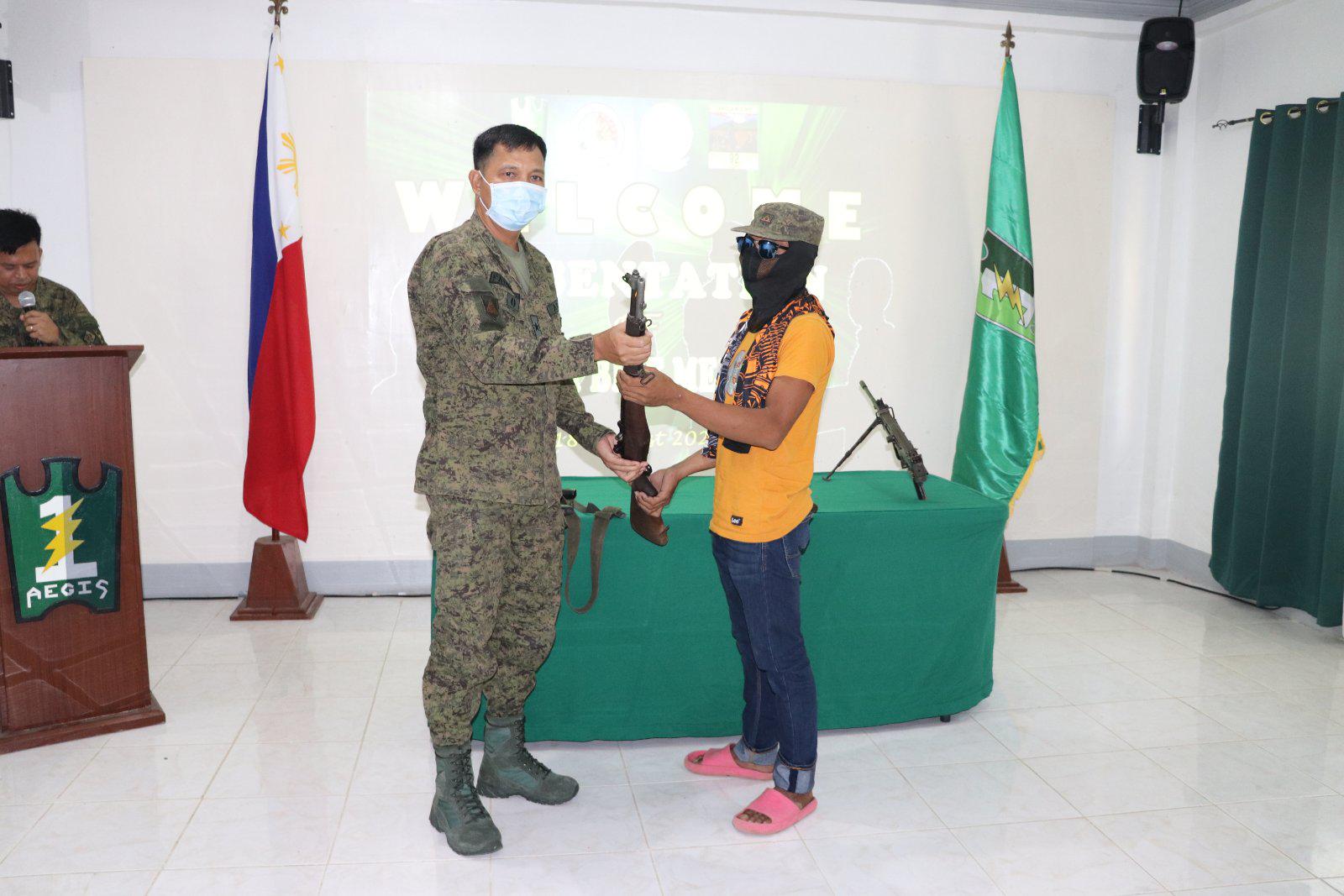This photograph captures a military enlistment or commencement ceremony set in what appears to be a government building, featuring a white tile floor and green curtains on the right-hand side. Dominating the scene are two primary figures centered in the image. On the left, there stands a soldier clad in gray and greenish jungle camouflage with combat boots, a white disposable face mask, and short black hair. He sports a patch on his right arm and appears to be handing over, or sharing, a rifle with a younger individual on his right. This second person, seemingly a civilian, is conspicuously dressed in casual attire: a yellow T-shirt, blue jeans rolled up at the cuffs, pink sandals, a camo hat matching the soldier's uniform, a black face mask covering his lower face, and sunglasses. They both grasp the rifle alternately, their hands interlocking along the weapon.

In the background, a green tablecloth-covered table holds another rifle. Two flags stand out prominently; one is blue, white, and red with a yellow symbol, while the other is green with a lightning bolt motif. On the left side of the image, behind a podium bearing the insignia "1-AEGIS" with a lightning bolt, a third individual, also in military attire, speaks into a microphone, indicating the ceremony's formal nature. A projector screen partially visible behind the trio features the word "Welcome," hinting at a welcoming event, possibly for new recruits or alliance. The context, combined with the attire and setting, suggests this is not a U.S. ceremony but rather from another country, potentially in Asia.